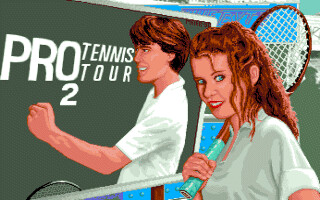This detailed rendering resembles a storyboard still for an advertisement pitch. The most prominent figure is a red-headed woman with long, flowing hair and striking turquoise eyes. Her lips are a vivid red-orange, and her white teeth and one ear are visible, emphasizing her confident smile. She wears a white short-sleeved shirt and casually carries a tennis racket over her shoulder, which features a distinctive brown and turquoise design. 

Beside her stands a billboard showcasing a male tennis player. He has brown hair and is also dressed in a white short-sleeved shirt. His right hand is clenched into a fist, exuding determination. The billboard text, written in bold white font, reads "Pro 2 Tennis Tour." At the bottom of the billboard, a black tennis racket is prominently displayed, adding an extra element of focus to the tennis-themed advertisement.